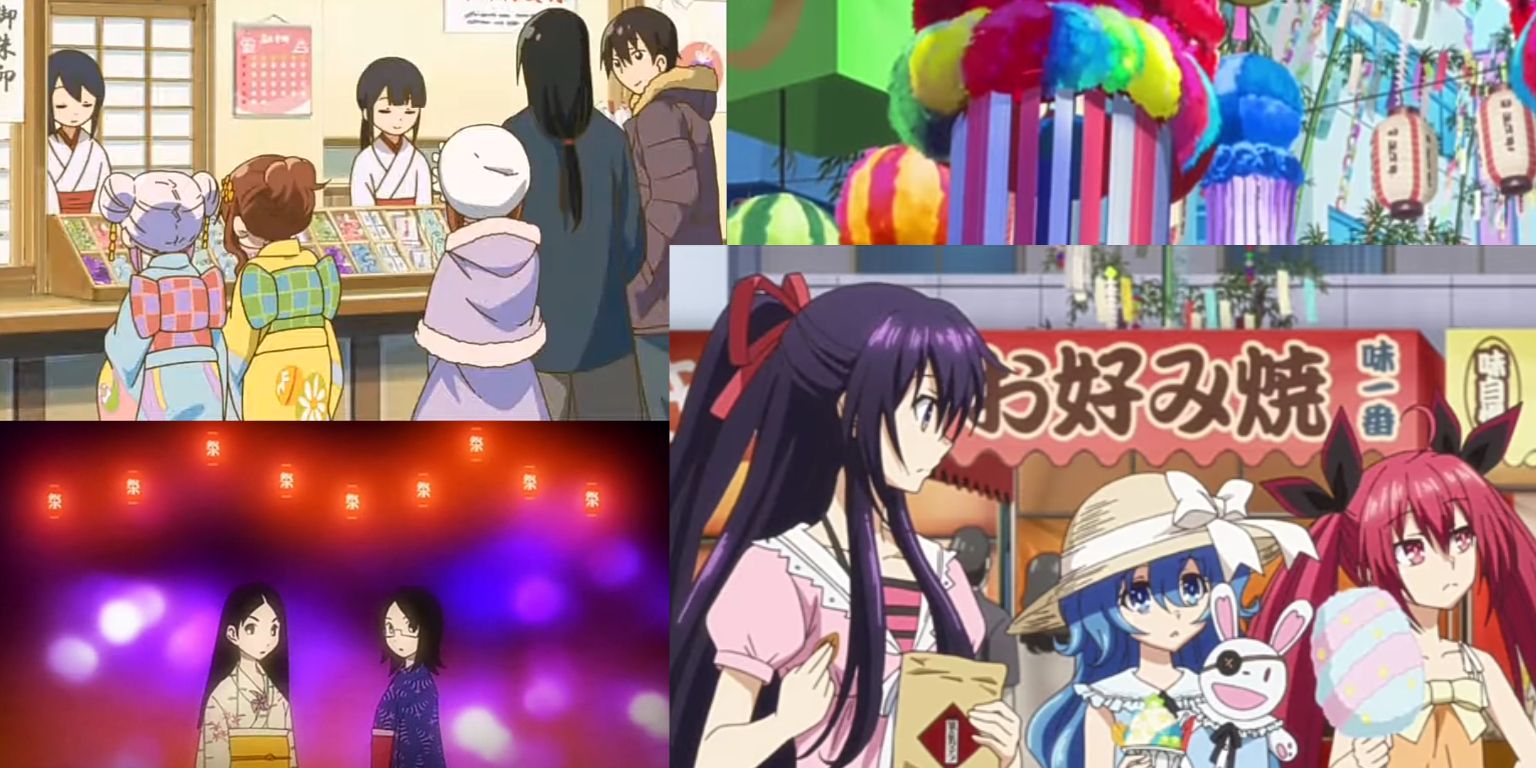This detailed rectangular collage features four distinct still shots from a Japanese anime. In the upper left-hand corner, five children are at a stall, seemingly at a candy store, with two Japanese women behind the counter, ready to serve them. The upper right-hand corner showcases vibrant street decor, including Chinese lanterns strung between buildings. In the lower left-hand corner, two Japanese women in kimonos stand facing each other, gazing off to the right, with purple and orange lights illuminating the scene above them. The lower right-hand corner, occupying a larger portion of the collage, portrays three girls walking through the street, each holding a different item: a brunette with a bag of chips, a blue-haired girl with a toy rabbit, and a redhead with cotton candy. The image is lively with festive lights and captures a busy, colorful street scene rich with cultural elements and youthful energy.